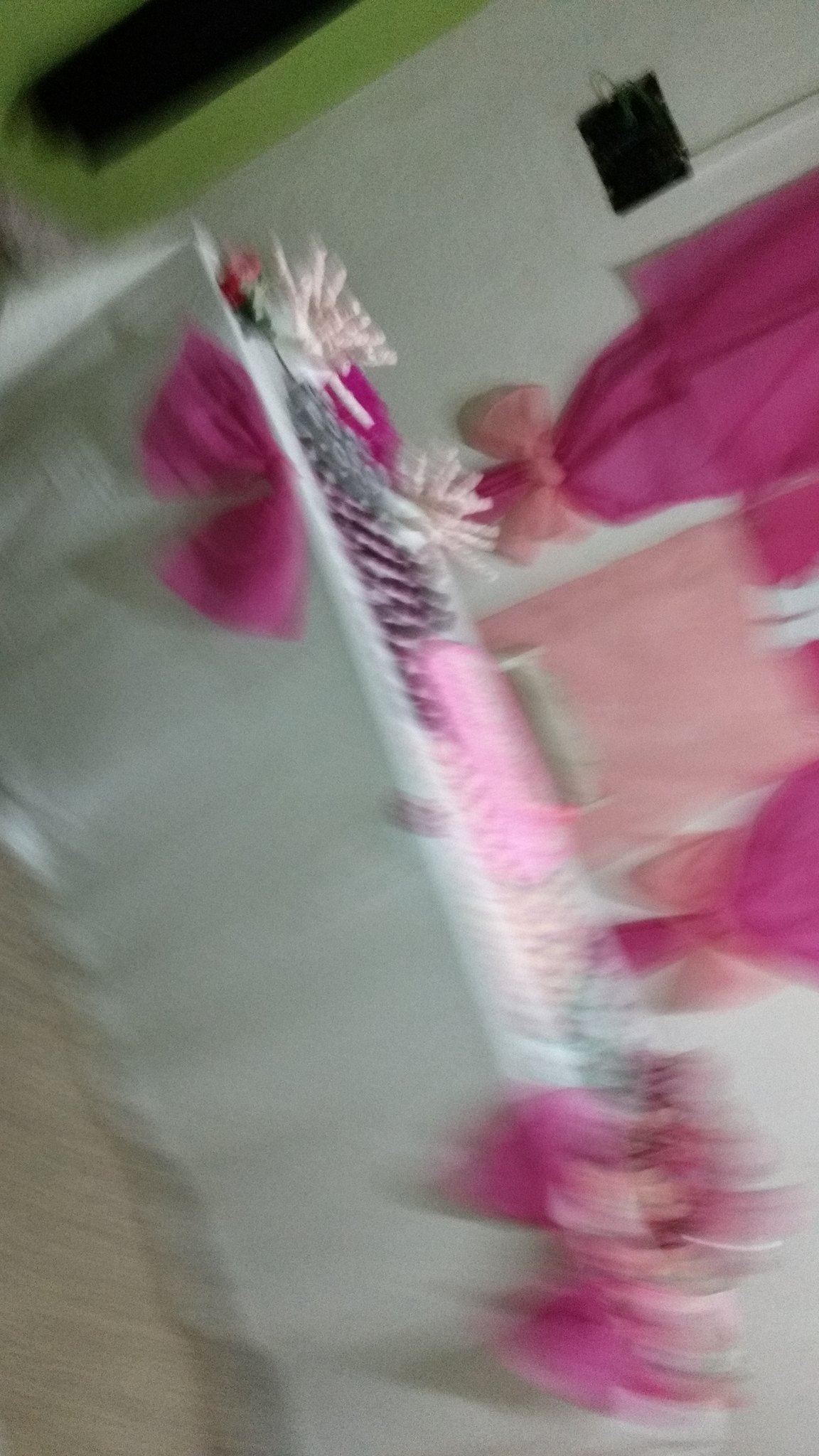The image is quite blurred, making the details somewhat difficult to discern. However, it features a green wall adorned with a black holder. In the foreground, there is a table draped in white fabric, accentuated with large pink bows. Behind the table, a white wall is visible, featuring a black square panel with wires extending from it. To the right, an opening with bright pink curtains tied back with matching pink bows adds a splash of vibrant color. The table appears to be laden with gifts, including one wrapped in black and white stripes and others in pink, all adorned with small white bows.